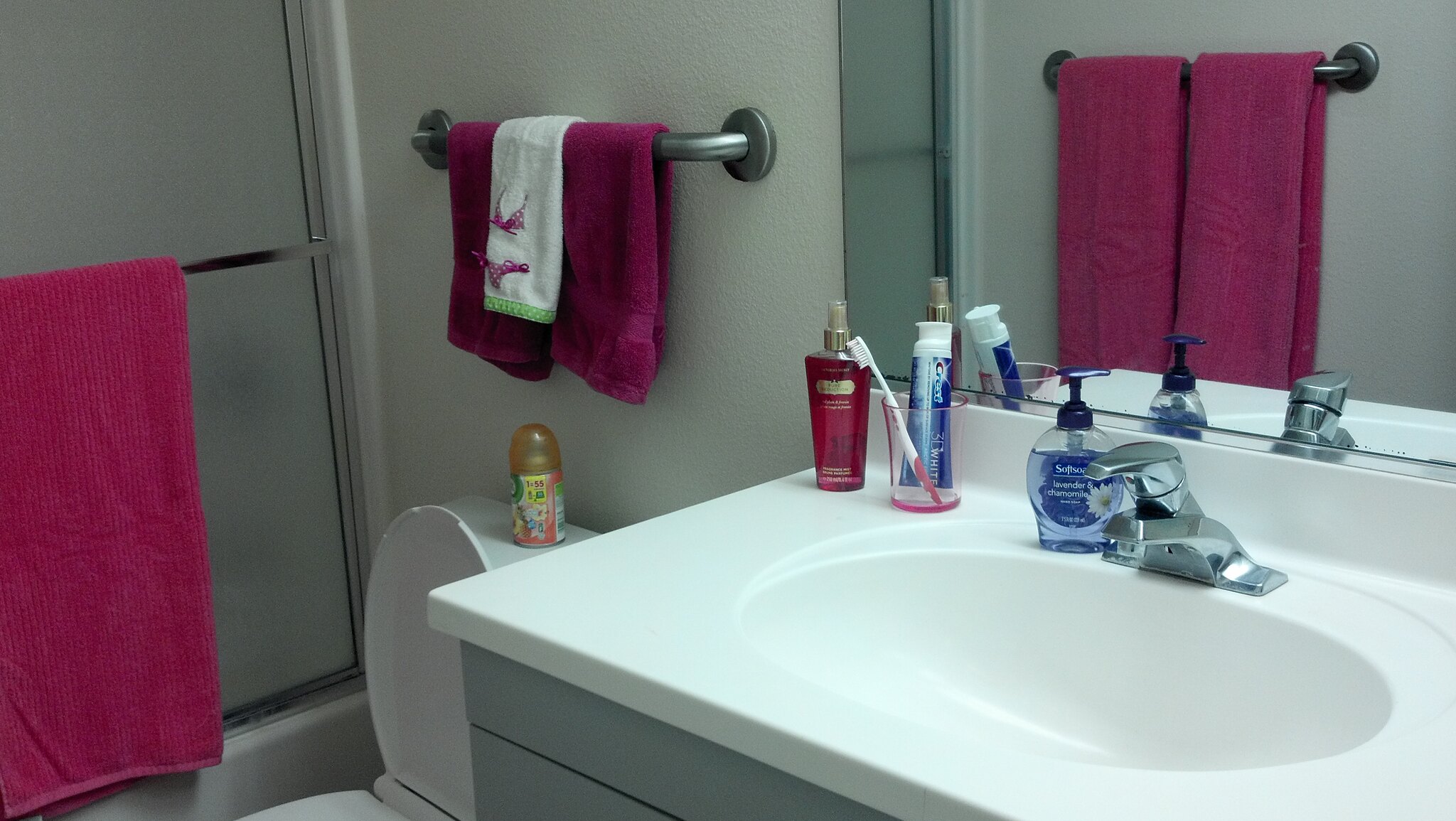The image showcases a neatly arranged bathroom. On the left side, a glass shower door features a bar with a pink towel hanging from it. Partially visible behind the door is the top of a toilet, adorned with an orange object marked with a colorful label in hues of blue, green, and red. Adjacent to the toilet is a towel rack holding three towels: two are solid red, while the third is white with red accents and green trim around the edge.

The sink area is pristine with a white countertop and basin. Atop the sink, there is a jar or bottle filled with a red fluid, distinguished by a gold patch and a silver cap. A glass positioned nearby contains a toothbrush, and there is also a tube of toothpaste and a pump dispenser with soap. Behind the sink, a mirror reflects the countertop and its items, including the faucet. Additionally, the reflection reveals two more pink towels hanging in the background.